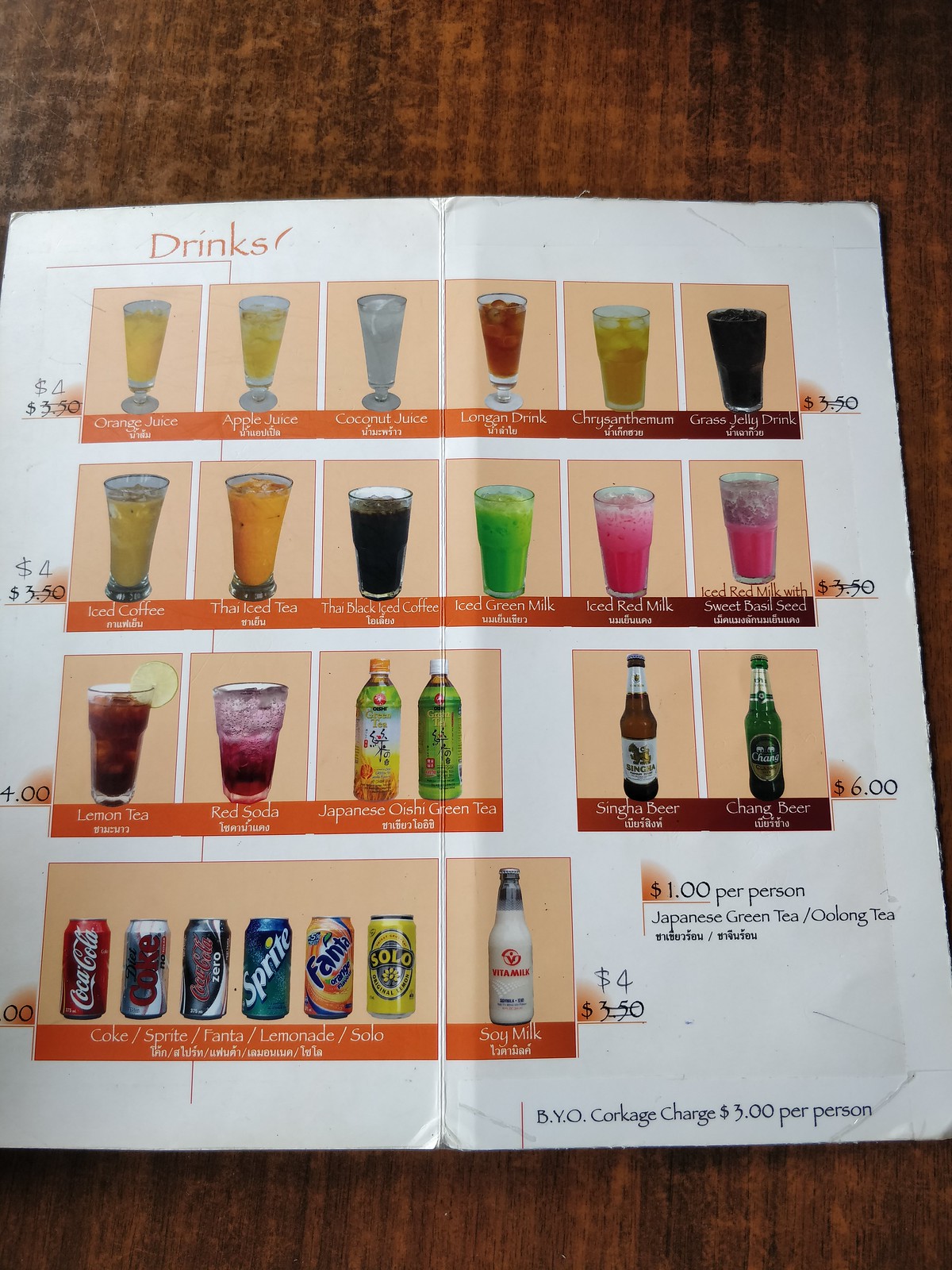This detailed image is of a menu presumably written in Japanese, featuring an assortment of beverages. The items are displayed methodically with prices and photographs. Notably, the menu includes an array of drinks such as orange juice, apple juice, coconut juice, longan drink, chrysanthemum drink, and grass jelly. The initial price of $3.50 for these drinks is crossed out and updated to $4.00. 

Another row showcases images set against a plain beige background featuring iced coffee, Thai iced tea, a black coffee variant, and iced green tea, amounting to six images in total. There is also a section including lemon tea, red soda, Japanese oshi, and green tea. Adjacent to this section, there is a blank space, followed by a selection of two different beers priced at $6.00 each. 

At the bottom, the menu displays a row of canned beverages alongside a bottle of soy milk, each listed for $4.00. Additionally, the menu highlights that Japanese green tea is available for $1.00 per person, with a noted corkage charge of $3.00 per person.